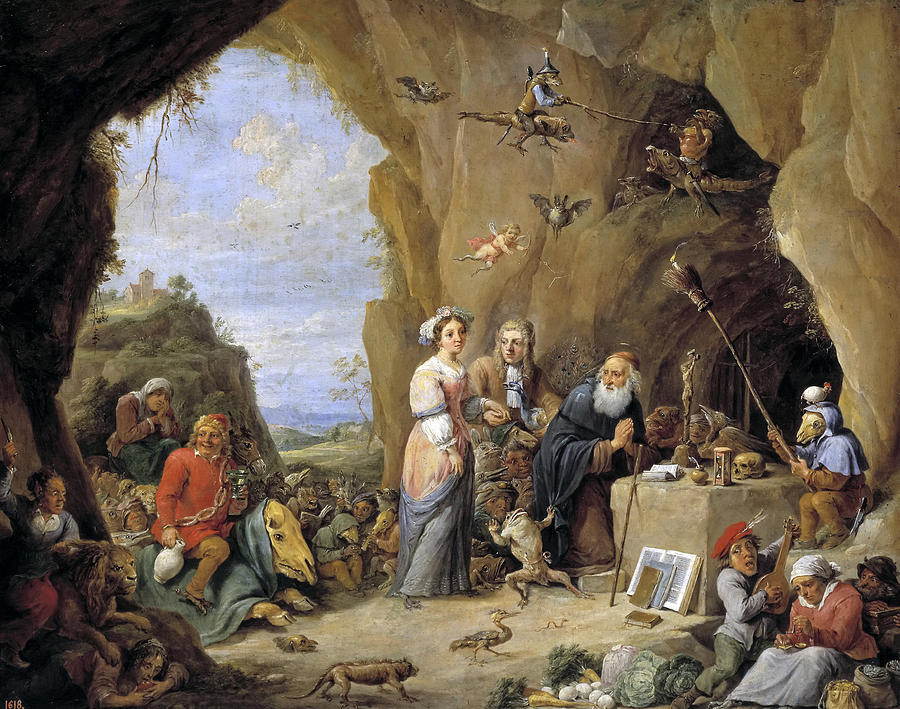This captivating painting, likely set in the 18th century or earlier, depicts a bustling, fantastical scene just inside the mouth of an expansive cave. Against the backdrop of mountains and a partly sunny blue sky, a collection of vibrant individuals and peculiar creatures engage in a variety of activities. On the left, a woman in a red shirt, grey pants, and white headdress sits serenely, listening to a man in grey attire and a beret, who is playing a lute. Nearby, an elderly man, identifiable by his white beard, moustache, and Jewish skullcap, stands at an altar with praying hands. The altar is adorned with a skull, a vase, and an open book, while a frog clings to his robe.

In front of the altar, another person, wearing a donkey mask and a blue cape, holds a pole, possibly an incense holder. Behind this assembly, a man dressed as a gentleman, complete with a white wig and a brown coat, clasps the hand of a woman in a striking white, orange, and grey dress with a matching headdress. Above this scene, a monkey riding a lizard wields a stick at another creature atop a lizard. 

In the middle of the foreground, a duck and a small four-legged animal can be observed moving leisurely. Nearby, a man in a red coat is seated atop what appears to be a cow draped in a grey blanket, holding a jug. Behind him, a woman stands with hands in prayer, gazing intently at the man. The bottom left corner features a striking image of a black man alongside some lions, adding to the scene's exotic and timeless feel.

The vivid painting is teeming with mystical and whimsical elements, including dancing frogs, strange critters, and wizard-like characters, creating a complex tapestry that evokes both biblical and fantastical themes in a surreal, picturesque outdoor cave setting.